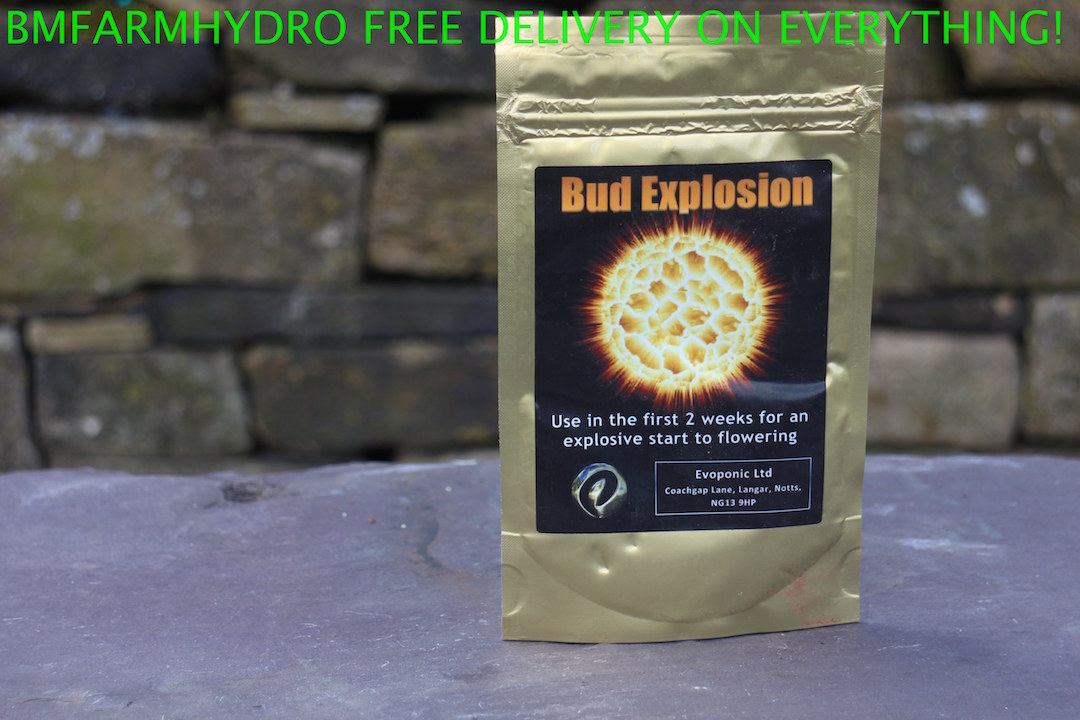The image is a promotional advertisement featuring a gold-colored, resealable plastic package labeled "Bud Explosion." The package, designed for use in the first two weeks to kickstart flowering, prominently displays a sticker with an image of an exploding sun or fiery ball. The sticker also includes the text "Bud Explosion" and the instruction, "Use in the first two weeks for an explosive start to flowering." Below the text, the company name and address are listed as "Evoponic Ltd, Coach Gap Lane, Langar, Knots, NG13 9HP." Additionally, the logo of the company appears in the bottom left corner of the sticker. The package is posed on a stone surface with a brick or stone wall in the background, providing a rustic backdrop. Across the top of the image, white text in green letters reads, "BM Farm Hydro - Free delivery on everything!"